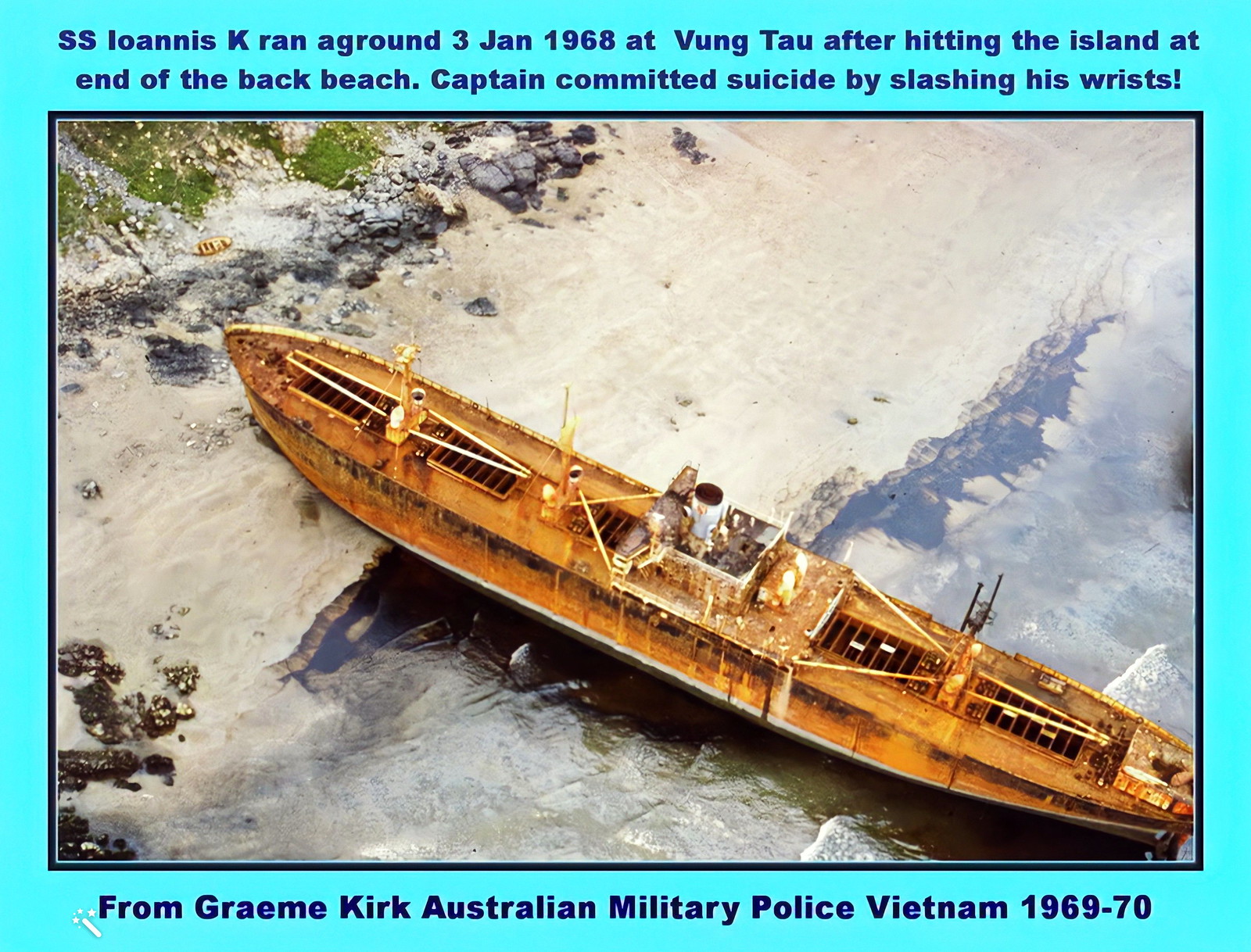The photograph, bordered in bright blue or turquoise, shows a large, rusty shipwreck marooned against a shoreline. The ship, identified as the SS Ioannis K., ran aground on January 3, 1968, at Vung Tau after hitting an island at the end of the back beach. The tragic scene captures the debilitated vessel thrust upon the sand, surrounded by some rocks and sparse grass. In the bottom right corner of the image, there’s a glimpse of water while the upper left side highlights the shore. The top border of the photograph has text in blue that details the ship's demise and the captain's suicide by slashing his wrists. Beneath the image, the bottom border includes a caption reading, "From Graham Kirk, Australian Military Police, Vietnam 1969-1970," providing context to this somber historical moment.